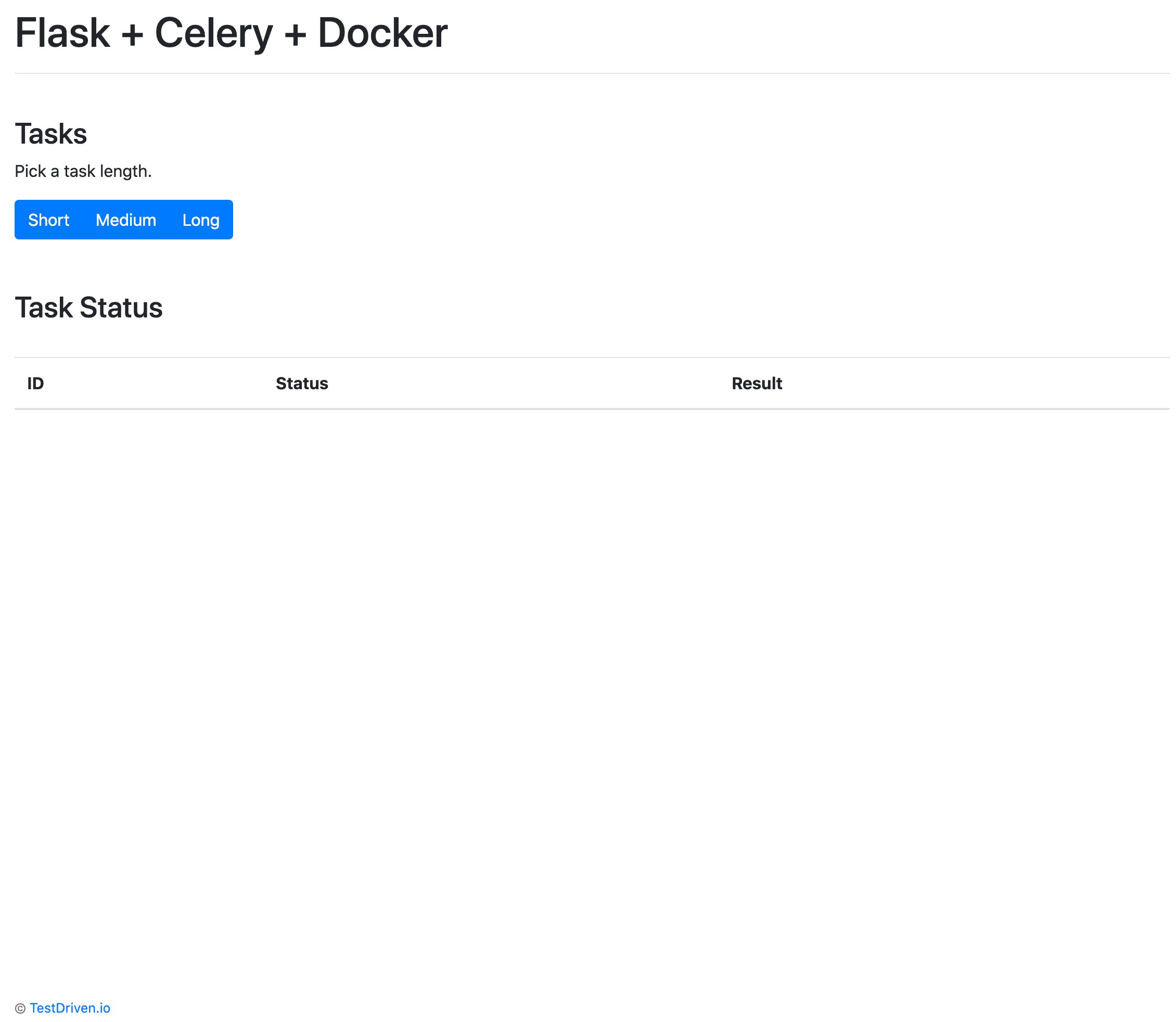In the upper left-hand corner of the photo, there are the words "Flask", "Celery", and "Docker" displayed in black font, each word starting with a capital letter. A thin gray line separates this section from the one below. In the lower section, there is some spacing followed by the word "Tasks" in black font with a capital T, although the font size is slightly smaller compared to "Flask", "Celery", and "Docker". Below "Tasks", in even smaller black font, is the phrase "Pick a task length." 

Beneath this phrase, there are three options displayed within blue boxes, each with white font, labeled "Short," "Medium," and "Long." Following this, the text "Task Status" appears. Below, a bar is presented with three labels: "ID," "Status," and "Result".